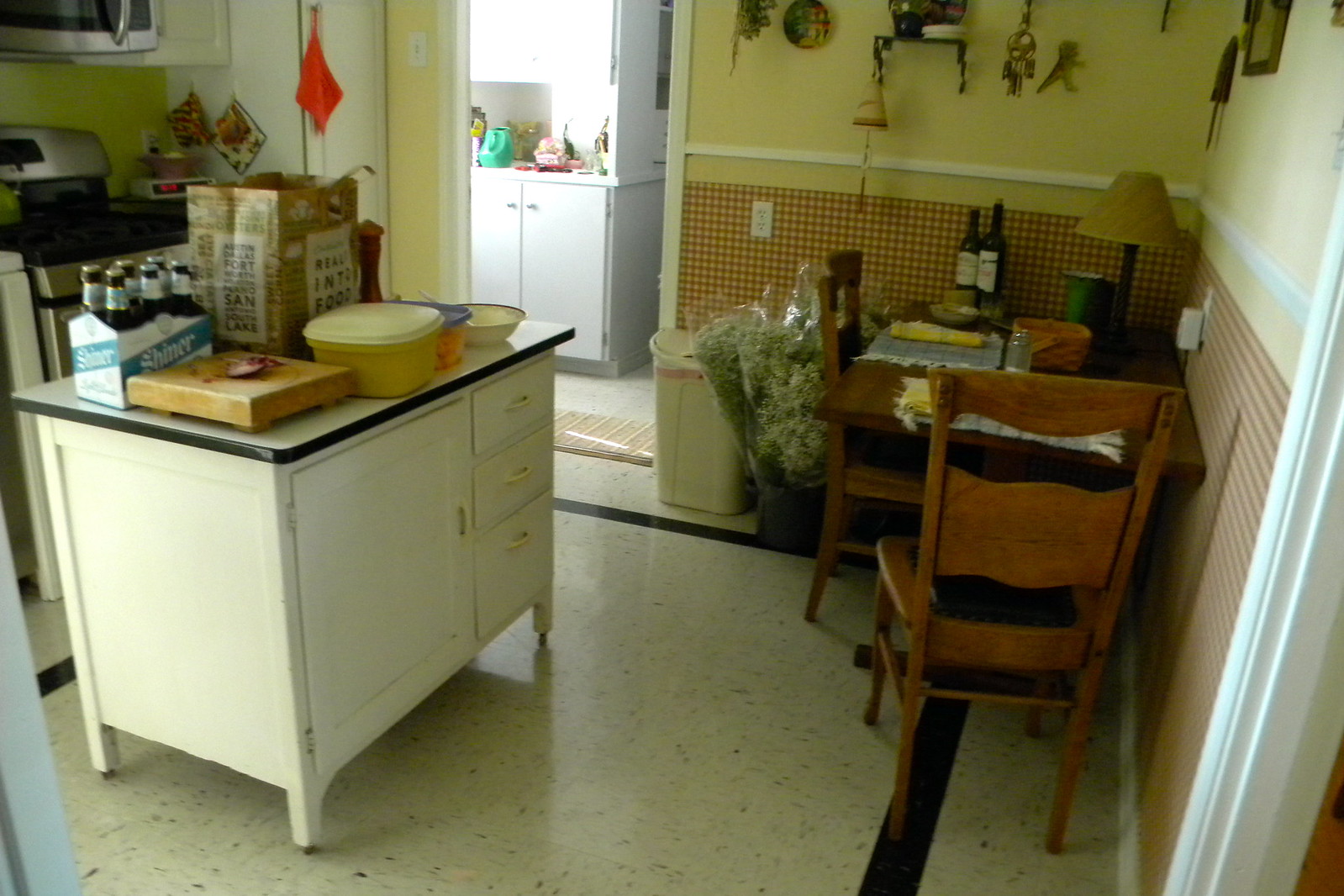The image depicts a small kitchen characterized by its white tile flooring bordered with black trim. The tiles are arranged in small squares, each with subtle white patches. Dominating the center of the kitchen is a white table featuring three drawers on the left side and a four-corner square door. The tabletop has a black outer line and a white center. 

Atop the table, several items are neatly placed: a yellow container, a clear container with a blue lid, a white plate, and a box of beers that is white with a blue sash. Behind the table, there are two boxes resembling cereal boxes. 

In the background, a stove is visible with a microwave mounted above it. Adjacent to this setup is a white cupboard situated in the corner of the room, which also contains a white-orange leg. A door is present, opening to what seems to be another kitchen. 

To the right is a cream-colored bin. The kitchen walls are adorned with wallpaper composed of a pattern of brown, grey, and cream squares. A smaller brown table with accompanying chairs sits against the wall, with three bouquets of white lilies positioned behind it. Additionally, two wine bottles are on the table, accompanied by a lamp on the far right. The table is set with cloths, suggesting it is ready for two diners.